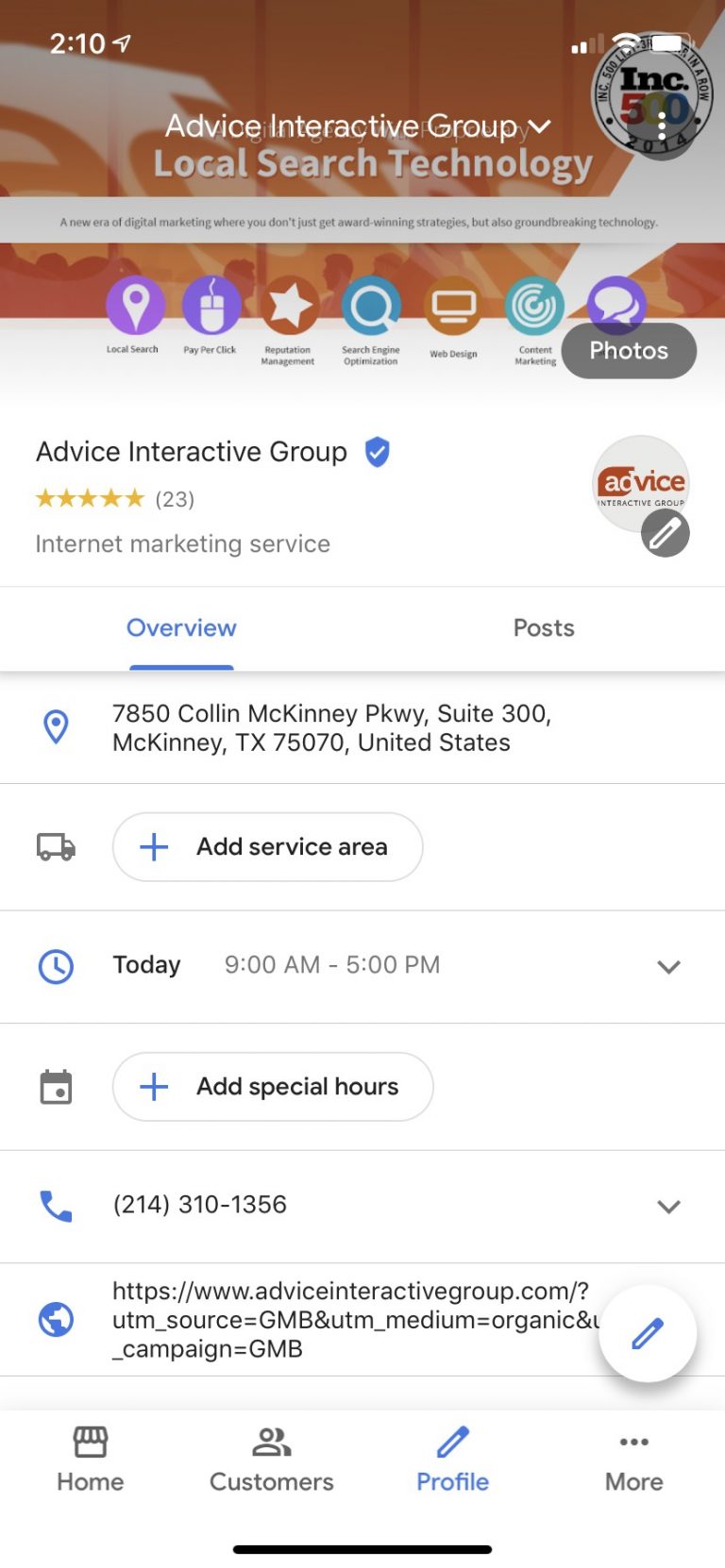The screenshot, captured on a smartphone, displays a variety of details. At the top left corner, the time is shown as 2:10, and to the right, there are indicators displaying 2 out of 4 bars of cellular signal, a full Wi-Fi signal, and an almost full battery icon. 

Centrally aligned below this, the text "Advice Interactive Group, Local Search Technology" is prominently featured. Beneath this heading, there is a row of icons, although their small, blurry nature makes them difficult to discern clearly. The icons appear to represent various functions: a pinpoint, a mouse, a star, a magnifying glass, a computer monitor, and a chat bubble.

Further down, it states, "Advice Interactive Group" has a 5-star rating from 23 reviews, qualifying it as an internet marketing service. To the right, the word "Post" is displayed, while on the left, there's "Overview" in blue, underlined hyperlink text.

At the very bottom, the address is listed as "7850 Collin McKinney Parkway, Suite 300, McKinney, Texas, 75070, United States." Below the address, there is an "Add Service Area" button.